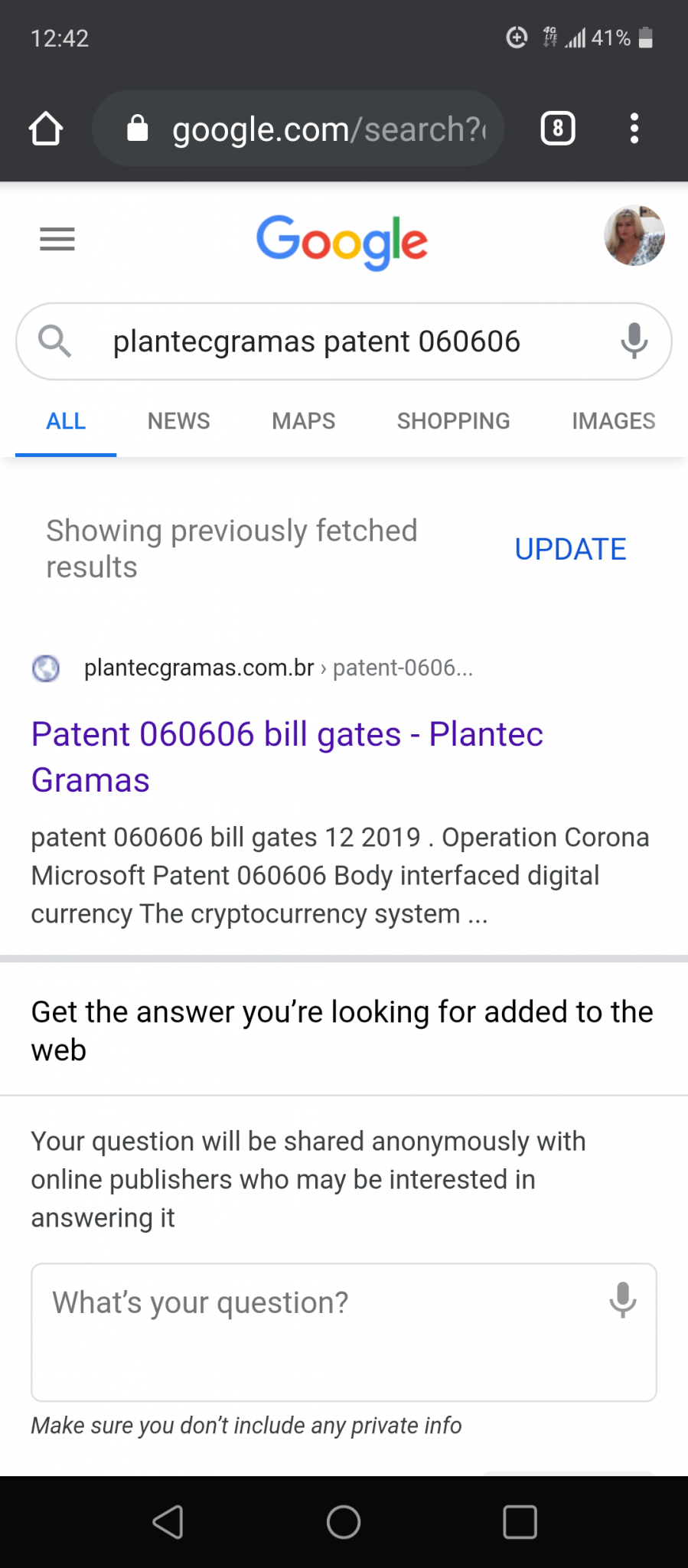The screenshot depicts a Google search interface on a mobile device. At the top, there's a black bar that displays the URL "google.com/search." Below this bar, the familiar Google homepage appears against a white background with the iconic "Google" logo centrally located. On the right side of the search bar, there is a round profile photo icon. The search query entered in the bar is "Plantagrammas patent 060606."

Underneath the search bar, there are navigation options labeled "All," "News," "Maps," "Shopping," and "Images." The page indicates it is showing previously fetched results for the query "Plantagrammas.com.br patent 060606." The first result mentioned is a link titled "Bill Gates, Plantek, Grommets, 12, 2019, Operation Corona, Microsoft Patent, Buddy, Interface, Digital Currency, the cryptocurrency system."

Further down, there is a horizontal line followed by the text: "Get the answers you're looking for added to the web. Your questions will be shared anonymously with online publishers who may be interested in answering it." Finally, there is a prompt asking, "What's your question?" accompanied by a cautionary note advising users to avoid including any private information.